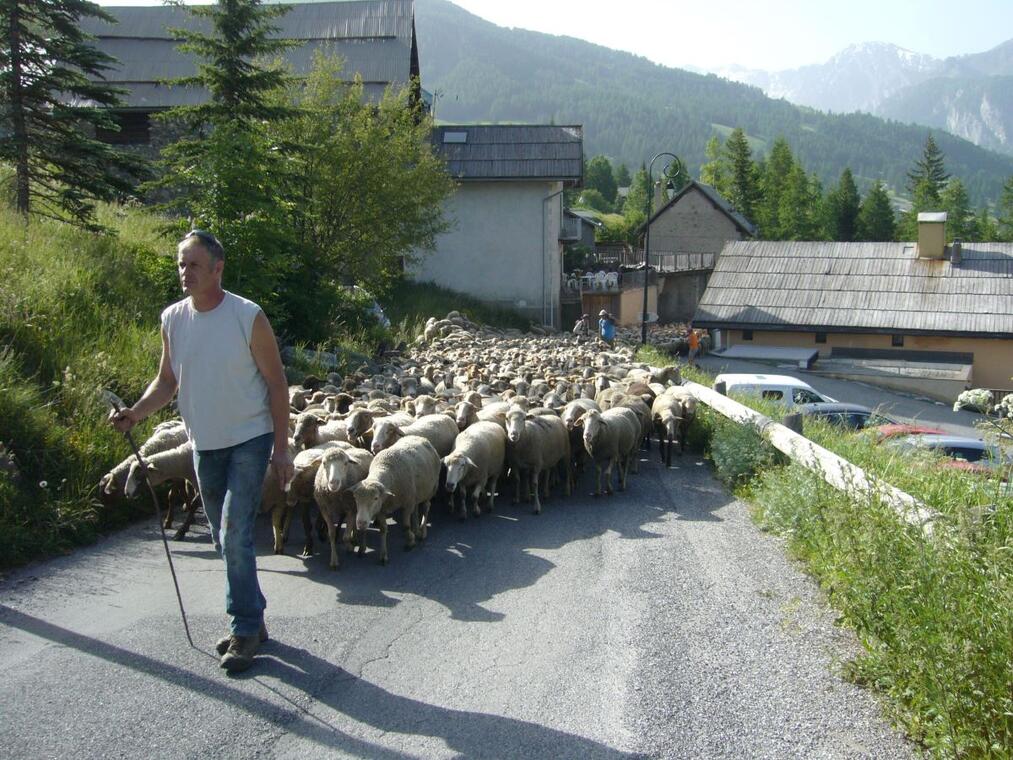In this picturesque European village, an older, gray-haired farmer, clad in a white sleeveless shirt, blue jeans, and boots, is depicted leading a vast, dense herd of grey and white sheep up a winding, paved road. The farmer, holding a walking stick with his right hand, guides the sheep from a parking lot at the village's edge, where a row of houses with thatched-style shingled roofs and sharp peaks are visible. The scene is awash with vibrant greenery; a grassy hill dotted with pine trees rises to the left of the road, while the village backs onto scenic mountain ranges with rocky, grey peaks. The vivid blue sky overhead indicates it is daytime. Scattered within the camera's view, at least 500 sheep densely crowd the road, stretching as far as the eye can see, while a few distant figures stand by, either waiting to pass or simply observing the pastoral procession.